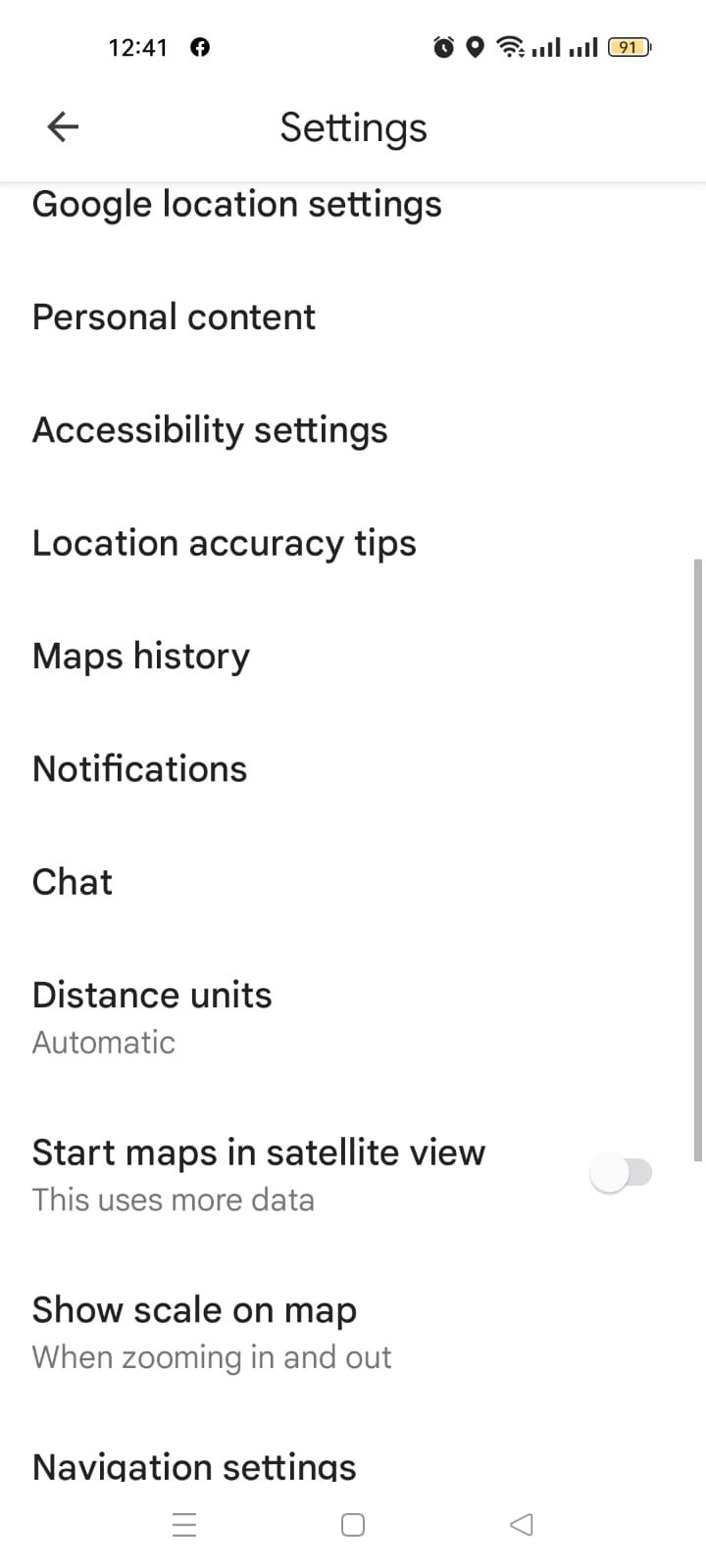This image depicts a screenshot of the Google Maps settings interface on a smartphone. The background at the top is white, showing a small black circle with an 'F' in it, along with the time "12:41." Below this, there is a left-arrow icon and a gear icon representing settings. A light blue line underscores the header text, which reads "Google location settings."

In the main content area, a series of menu options are listed:

- Personal content
- Accessibility settings
- Location accuracy tips
- Maps history
- Notifications
- Chat
- Distance units, currently set to "Automatic"
- Start maps in satellite view, with an additional note that this uses more data, accompanied by a white toggle switch
- Show scale on map when zooming in and out
- Navigation settings

A vertical blue line runs down the right side of the interface. At the bottom, standard navigation icons are visible: a circular home button, a three-line menu button, a square for recent apps, and a back arrow.

Overall, this image provides a comprehensive overview of various customizable settings in the Google Maps application on a smartphone.